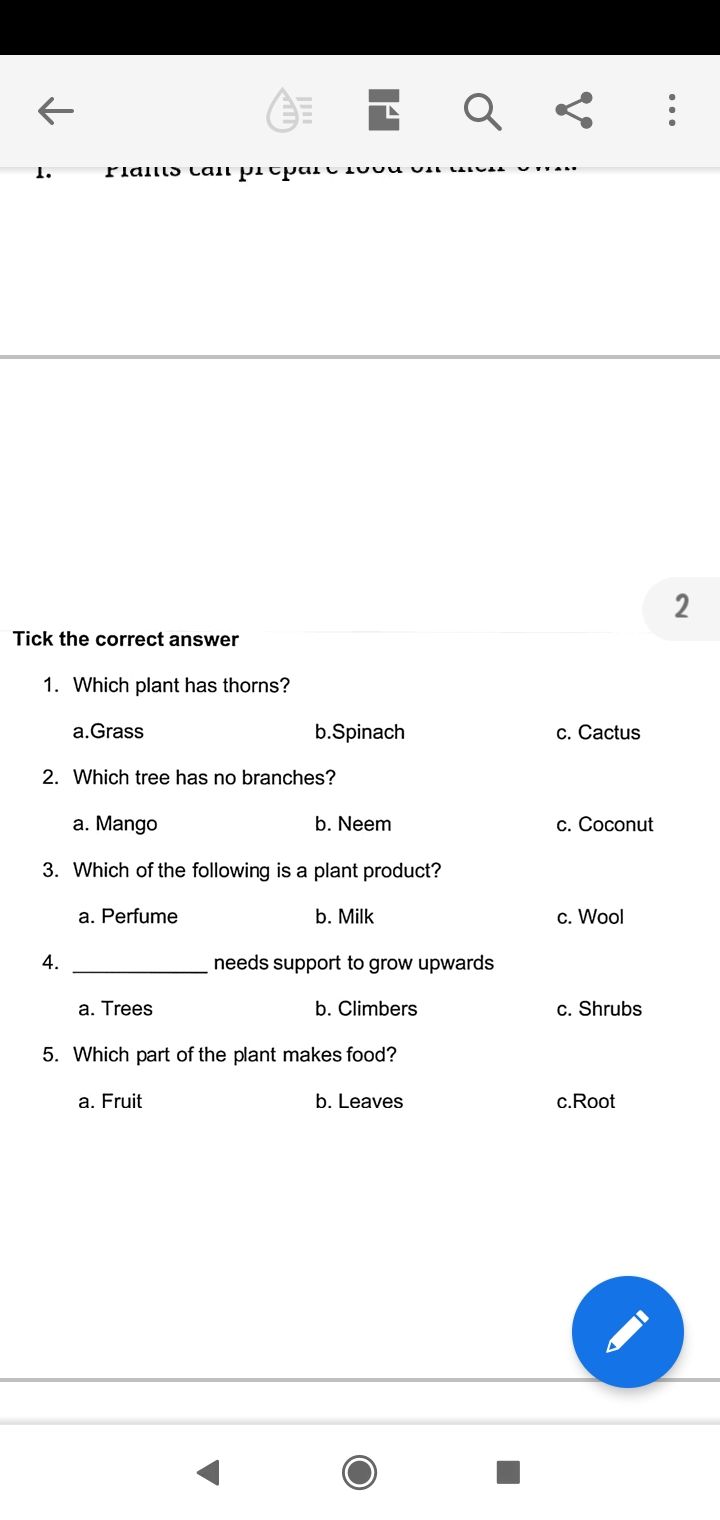In the image, a quiz interface on a website is displayed. The visible portion of the quiz begins with an incomplete first question that is only partially readable: "plants can prepare..." followed by a section under it instructing participants to "tick the correct answer." 

The multiple-choice quiz consists of five questions, each with three answer options:

1. **Which plant has thorns?**
   - A: Grass
   - B: Spinach
   - C: Cactus

2. **Which tree has no branches?**
   - A: Mango
   - B: Neem
   - C: Coconut

3. **Which of the following is a plant product?**
   - A: Perfume
   - B: Milk
   - C: Wool

4. **____ needs support to grow upwards.**
   - A: Trees
   - B: Climbers
   - C: Shrubs

5. **Which part of the plant makes food?**
   - A: Fruit
   - B: Leaves
   - C: Root

A small blue circle with a pencil icon appears at the bottom, presumably allowing users to add comments or notes.